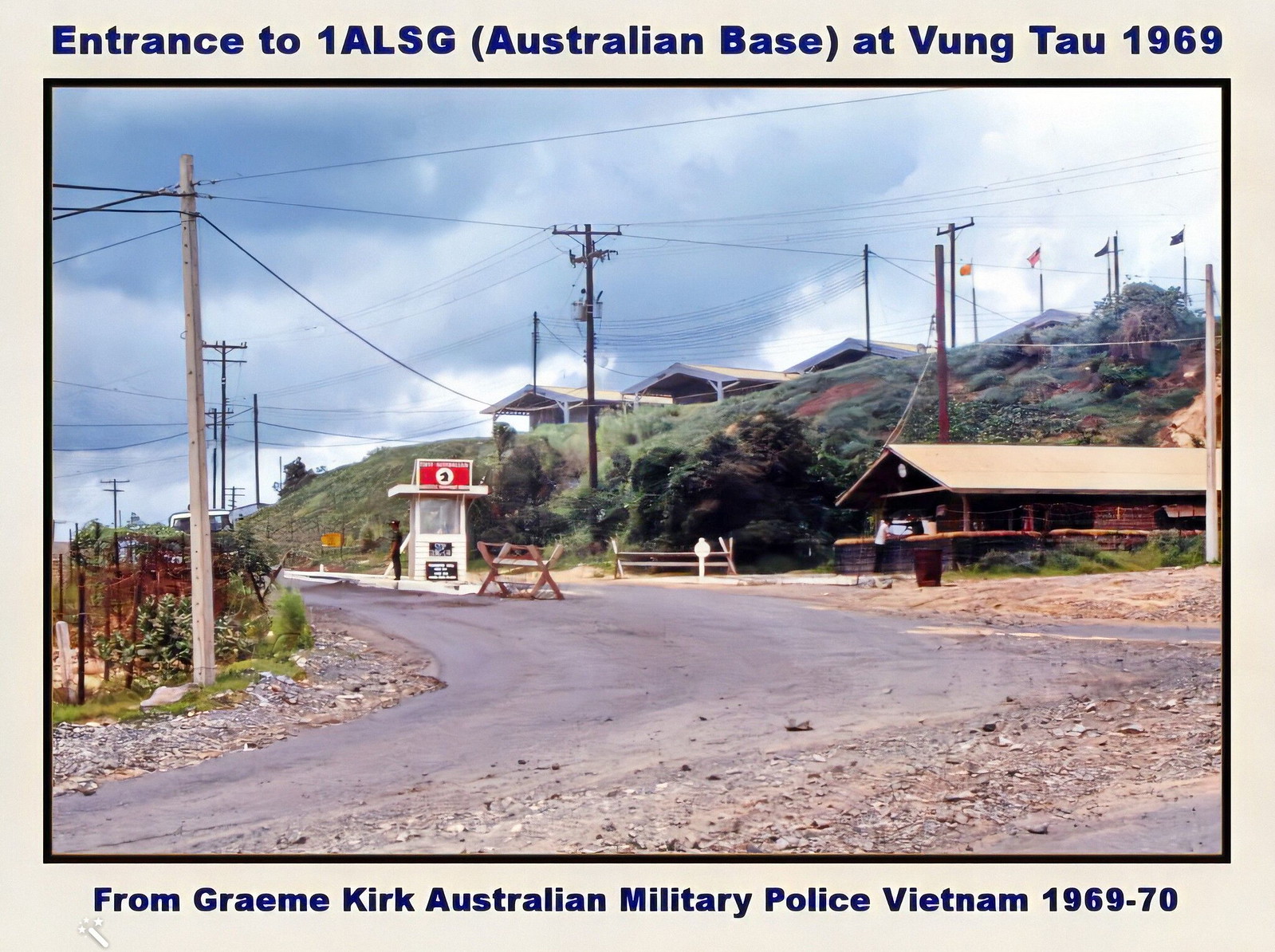The photograph captures an outdoor scene at the "Entrance to 1ALSG, Australian Base at Vung Tau, 1969," as stated in dark navy blue print on the top header of the gray border framing the rectangular image. A narrow black border further outlines the gray border. The caption at the footer reads, "From Graham Kirk, Australian Military Police, Vietnam, 1969 to 1970." The sky dominates the top half of the image, transitioning from dark grayish-blue clouds on the left to a lighter gray towards the upper right corner. Below the sky on the right-hand side, there is a green grassy hill where bits of rooftops and flags, including an American flag, peek out at the top. At the base of the hill lies a paved road with a guard station manned by a guard. Surrounding the road and station are long power poles with lines crisscrossing above, and various rocky patches on the ground. A cabin is visible to the right side of the image, amidst abundant trees and bushes.